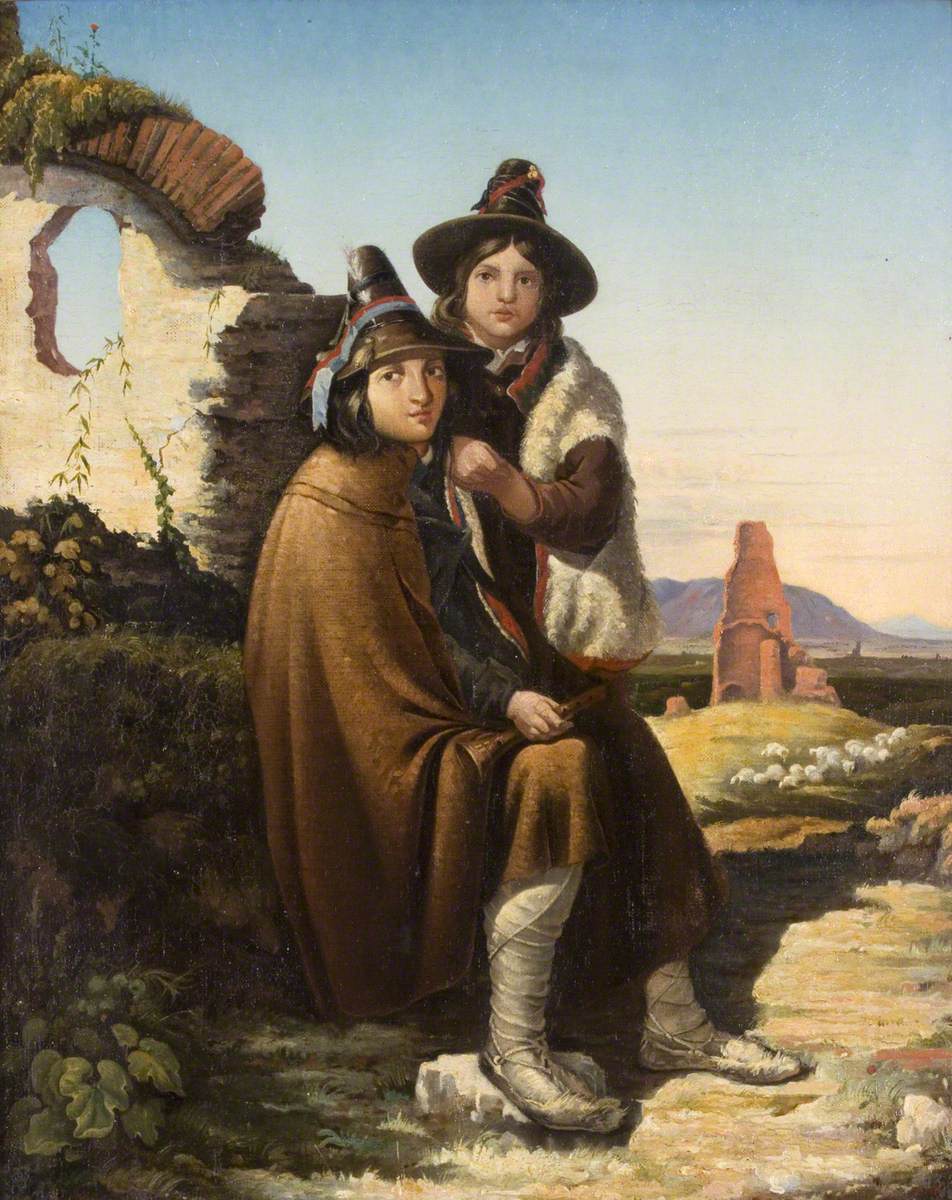This detailed painting depicts two figures resembling pilgrims set in an outdoor scene during the daytime. The central figure, a young boy, is seated on a stone, dressed in a brown robe, a black hat adorned with a ribbon, and white shoes. He holds a musical instrument in one hand. Behind him stands a young girl, identifiable by her long, shoulder-length hair parted at the middle. She wears a black hat similar in style, a white fur coat over a brown shirt, and clasps the boy's shoulder. The pair are situated next to a dilapidated white wall with a hole in it, around which vines and plants intertwine. The ground is a blend of cream, white, and green hues, adorned with small greenery and leaves. Further back, another broken structure painted brown can be seen, leading up to a hill and a yellow sky in the background. The painting is in portrait orientation, capturing an intricate mix of colonial attire and a rough, overgrown landscape.